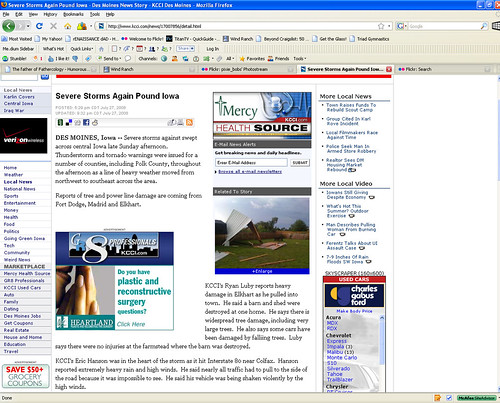The image features an exceptionally old version of Mozilla Firefox, identifiable by its dated interface and excessive clutter. The browser's title bar reads "Severe Storms Again, Pound Iowa, Des Moines Stories, Casey J. Malone's Mozilla Firefox," suggesting it predates modern web layouts.

The browser's toolbar is overloaded with numerous add-ons and widgets, to the point of resembling the overly customized browsers sometimes found on elderly relatives' computers. The visible webpage is a news site, albeit hard to discern due to graininess, which reports on severe weather events in Iowa. It shows a headline about destructive storms in Des Moines.

Ad banners are liberally sprinkled across the page, testament to a time before effective ad-blocking extensions were commonplace. Multiple tabs are open, adding to the chaotic appearance. The overall aesthetic is a nostalgic but cluttered mess, highlighting the significant evolution of web browsers over the past decade.